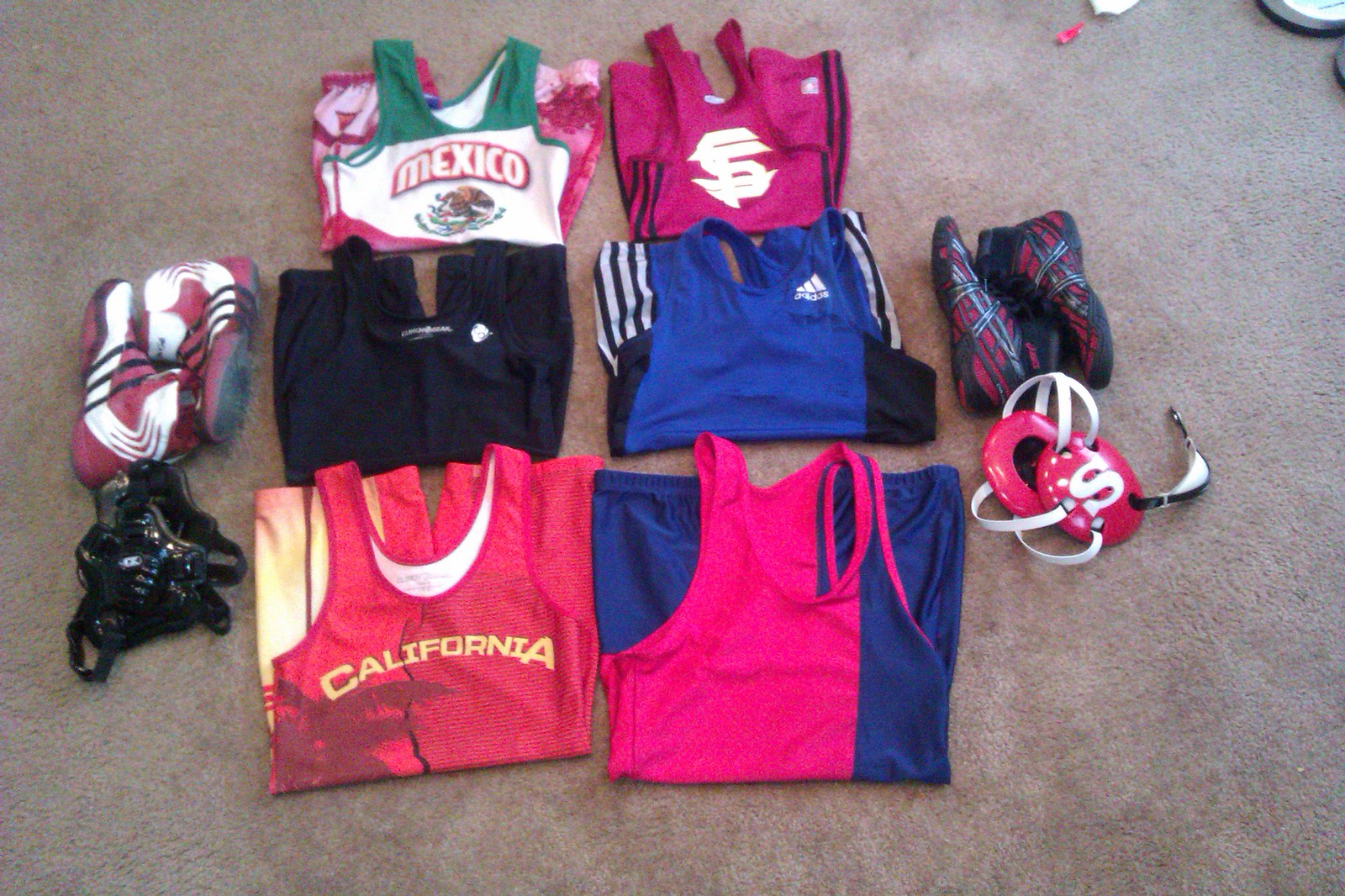The photograph is taken from above, showcasing a light brown carpet that serves as a backdrop for a neatly arranged collection of children's sportswear and accessories. On the carpet, there are six folded tank tops and matching shorts, each in a variety of vibrant colors including red, white, green, blue, yellow, purple, and pink. Some of these outfits feature distinct logos and team names, such as "California" and "Mexico," with one royal blue Adidas set that displays black and white stripes.

Towards the left side of the image, there's a pair of burgundy and white shoes, positioned near a small, unidentified black object which may be a piece of sports gear or padding. In the top right corner, another pair of shoes is visible; these are red with black and white plaid patterns. Positioned below this pair is an intriguing set of magenta-colored ear muffs with two connecting straps, which might include a mouth guard or chin guard as part of their design. This well-composed assortment of sports clothing and gear hints at an organized preparation for athletic activities.